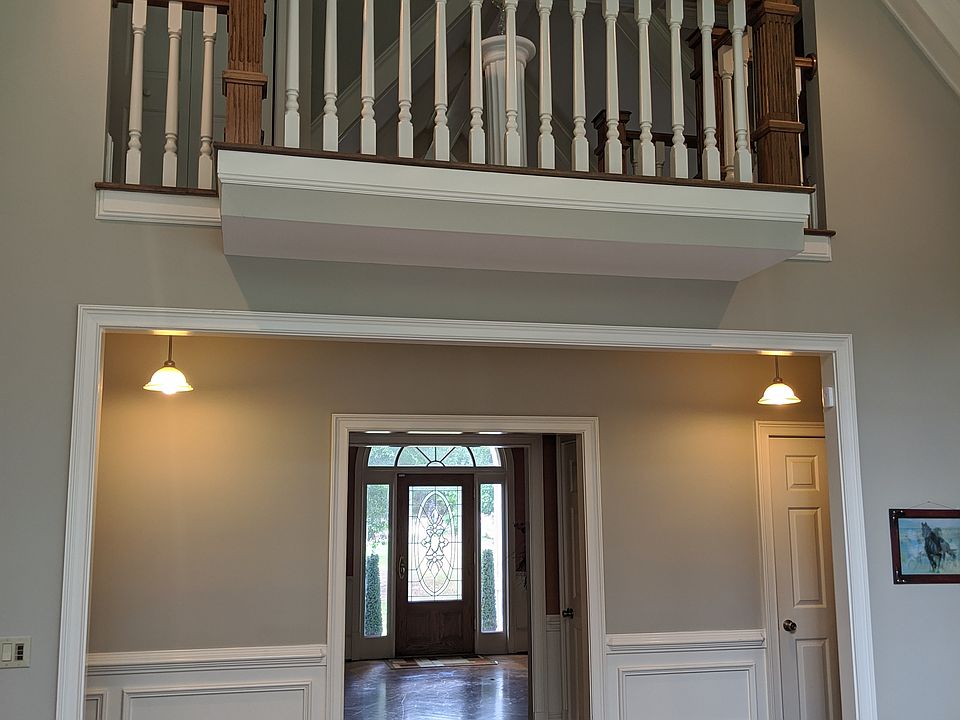The image captures the interior of a beautifully designed residential house, viewed from a central living area towards the front entrance. A large white doorway opens into a stylish hallway, meticulously adorned with gray walls and accented with white wainscoting and detailed molding. The hallway showcases hanging lamps adding to the elegant ambiance. At the far end, a glass-paneled front door, framed by tall windows and glass panels, features a semi-circle window above and intricate stained glass work. Flanking the front door, tall trees are visible from outside. On the upper level, above the main doorway, a small balcony with white spindles protrudes from the wall, adding a touch of sophistication. This balcony houses a large white pedestal with a statue on top, epitomizing classic architectural elegance. A photograph in a brown frame, depicting a gray animal, hangs to the right, further enhancing the décor. The dominant colors in the image are white, gray, brown, and tan, creating a harmonious and refined interior.